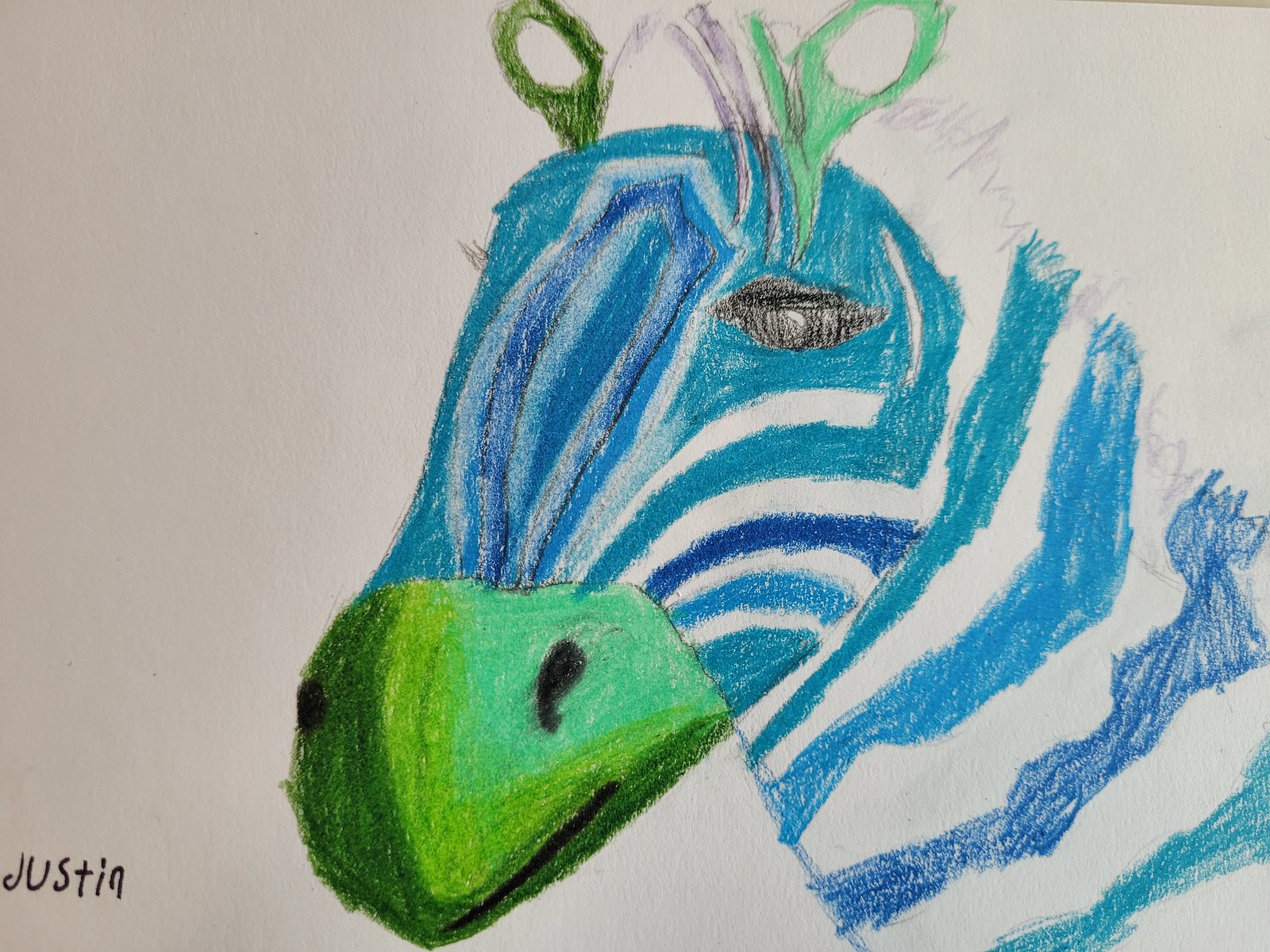This image showcases a vibrant drawing created using colored pencils, crayons, or possibly oil pastels. The artwork depicts a zebra on a white paper background that entirely fills the image's frame. Unlike a traditional zebra, this one features a creative twist with its stripes rendered in varying shades of blue—deep navy, medium indigo, light sky blue, and white.

The zebra’s snout and ears provide an additional splash of color, rendered in diverse shades of green. The eyes are filled in with black, as are the nostrils, adding a sense of lifelike detail. The head of the zebra is centrally positioned in the composition, capturing the top of its ears and extending down to about halfway along its neck, with the rest of its body extending beyond the border of the frame.

In the lower left-hand corner, the name "Justin" is penned in black ink, presumably the name of the artist. This imaginative and colorful rendition of a zebra breathes fresh life into a classic subject, drawing the viewer in with its unconventional use of color and detailed presentation.